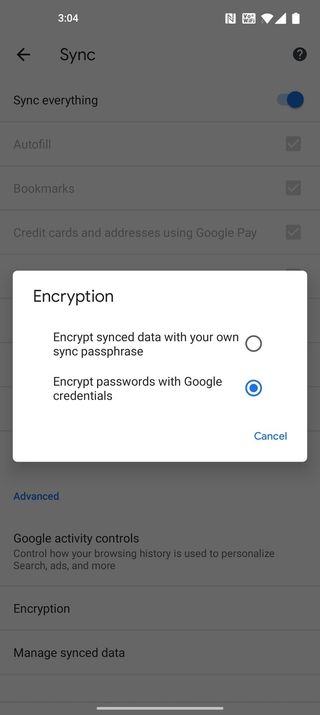The image appears to be a screenshot from a mobile device, primarily featuring a pop-up window related to data encryption settings. The majority of the background is grayed out, but it's still possible to discern some options pertaining to synchronization, like "Sync everything", "Autofill", "Bookmarks", "Credit cards, and addresses using Google Play", "Advanced Google activity controls", "Encryption", and "Manage synced data".

The focus of the image is a white pop-up window with predominantly black text, and some blue text for selectable options. The title of the pop-up is "Encryption". Below the title, there are two encryption options presented:

1. "Encrypt synced data with your own sync passphrase", accompanied by a circle for selection.
2. "Encrypt passwords with Google credentials", which has a blue circle with a blue dot, indicating it is currently selected by the user.

At the bottom of the pop-up, there's an option to cancel the action, indicated by the word "Cancel" in blue text.